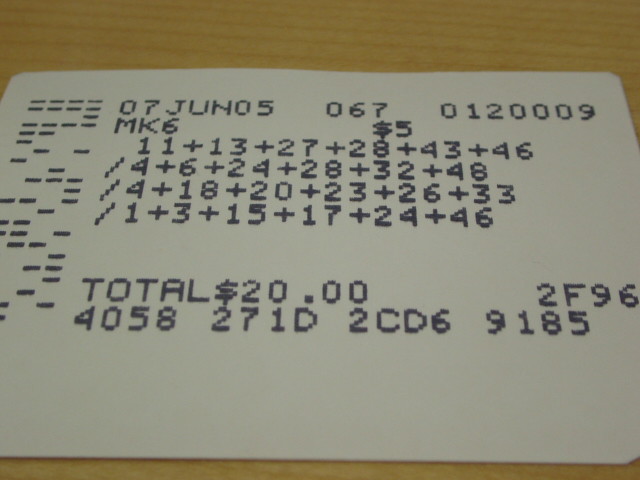The image features a single white rectangular object with rounded corners, resembling a ticket stub or receipt, prominently centered on a light wood grain table. The setting appears to be indoors. At the top of the ticket, the text reads "07 June 05," followed by an assortment of numbers and letters: "067 012 0009 MK6." Below this, there is a line indicating "$5," and then a sequence of mathematical additions such as "11 + 13 + 27 + 28 + 43 + 46," which extends over four lines. Towards the bottom, the ticket states "total $20," accompanied by a series of alphanumeric characters: "F9 6 4 0 5 8 2 7 1 D 2 CD 6 9 1 8 5." The ticket occupies almost the entire frame, and there are no other objects in the image. The color palette includes different shades of brown, white, and black.